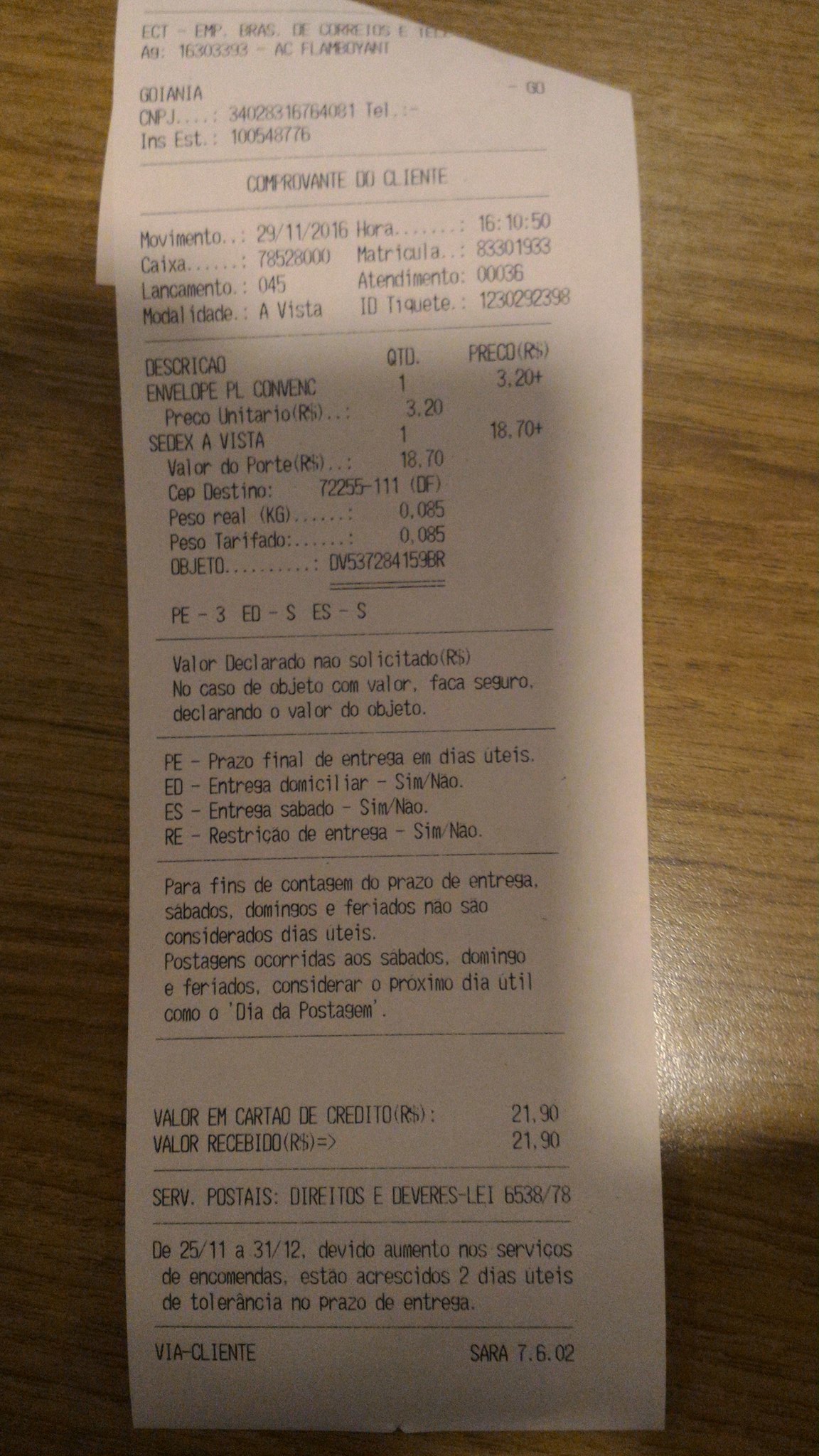This image features a slightly blurred, top-view photograph of a receipt, partially shadowed, and placed on a brown wooden surface, likely a table. The receipt is written in a foreign language, possibly Portuguese, indicating a purchase made on November 29, 2016, at 4:10:50 p.m. The document appears folded at the top, obscuring some details, but clearly shows text in black ink on white paper. It includes various items, such as an envelope, and mentions terms and codes related to payment methods and delivery options. The total amount spent is noted at 21.90, and the receipt indicates the use of a credit card for the transaction.